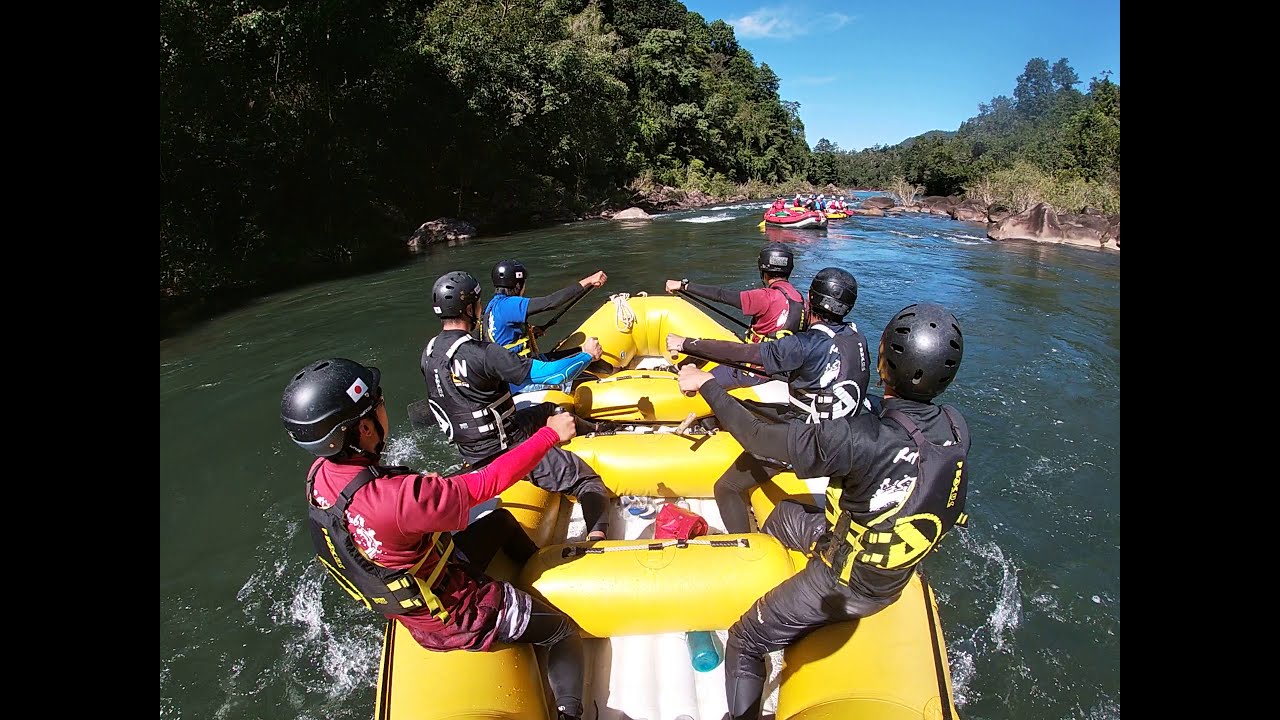In the picture, a group of people are engaged in whitewater rafting on a calm section of a greenish river surrounded by dense brush and tree-covered banks. The left bank features a steep, densely vegetated hillside, while the right bank is lower but equally covered in dense greenery. The clear blue sky above has a single wispy white cloud. There are several rafts on the river, predominantly red and yellow, with the scene focused on a yellow raft in the foreground and a red raft further ahead. The yellow raft in the center contains six people, three on each side, sitting on the edges and actively paddling with their oars to navigate the river. Almost all participants are wearing black helmets and life vests, while their shirts vary, with most in black and a couple in red. The group moves in a line, with rafts closely following one another, ensuring safety in numbers. Despite the calm water at this point, the persistence of their paddling indicates anticipation of more turbulent rapids ahead.